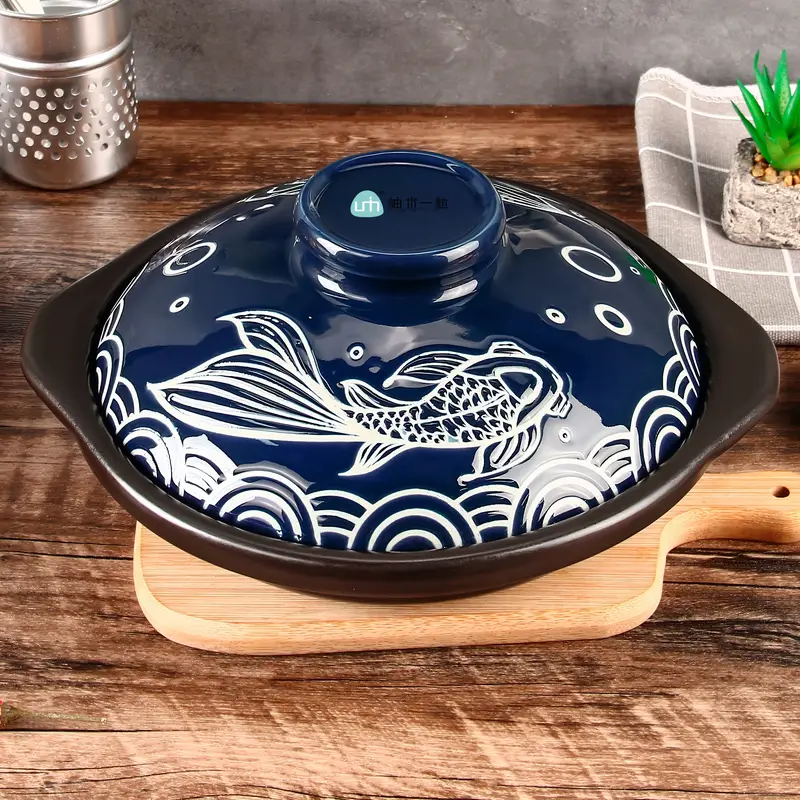The photograph captures a detailed and vibrant kitchen scene centered around a striking ceramic pot. The pot, used for Asian cooking, features a black, oval-shaped base with handles on either side, likely made of ceramic or metal. It has a shiny blue ceramic lid adorned with intricate white designs, including a swimming koi fish and a bubbles motif, creating a textured geometric pattern around the edge with rainbow-like arches and connecting lines. The lid also has a circular grip handle.

This pot is seated atop a wooden cutting board, itself resting on a wooden countertop. To the top left of the frame, a silver perforated container holds various utensils, while at the top right, a gray and white striped folded towel or washcloth supports a decorative succulent perched in a small pot with tiny pebbles. This arrangement creates a visually appealing and inviting kitchen setup, combining functionality with aesthetic touches.